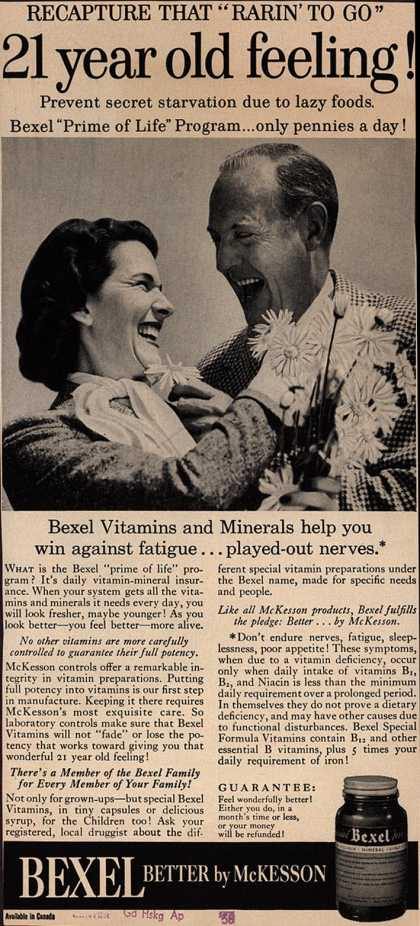In a retro newspaper advertisement styled in beige tones and Times New Roman font, an image of a joyous couple, possibly recently married, captures the essence of vitality and happiness. The man, appearing in his 40s or 50s, dons a plaid-patterned suit, with a beaming smile that suggests laughter. He embraces a woman, who wears a long-sleeved blouse paired with a light-colored scarf around her neck, her short, dark, curly hair framing a similarly joyous expression. She holds a small bouquet of daisies, her red-painted nails adding a splash of color to the black-and-white photo. The headline reads, "Recapture that rare 21-year-old feeling! Prevent secret starvation due to lazy foods."

An enticing tagline, “Bexyl Prime of Life program – only pennies a day!” promotes a daily routine of Bexyl vitamins and minerals said to combat fatigue, nerves, and other symptoms of nutrient deficiency. The ad highlights that Bexyl contains essential B vitamins, including B12 and niacin, as well as five times the daily requirement of iron. With bold claims and a money-back guarantee, Bexyl promises to make users feel “wonderfully better” or their money refunded. The photo and ad together portray a vibrant, youthful energy, suggesting that Bexyl is the secret to maintaining youthful vitality and combating the hidden dangers of inadequate nutrition from "lazy foods."